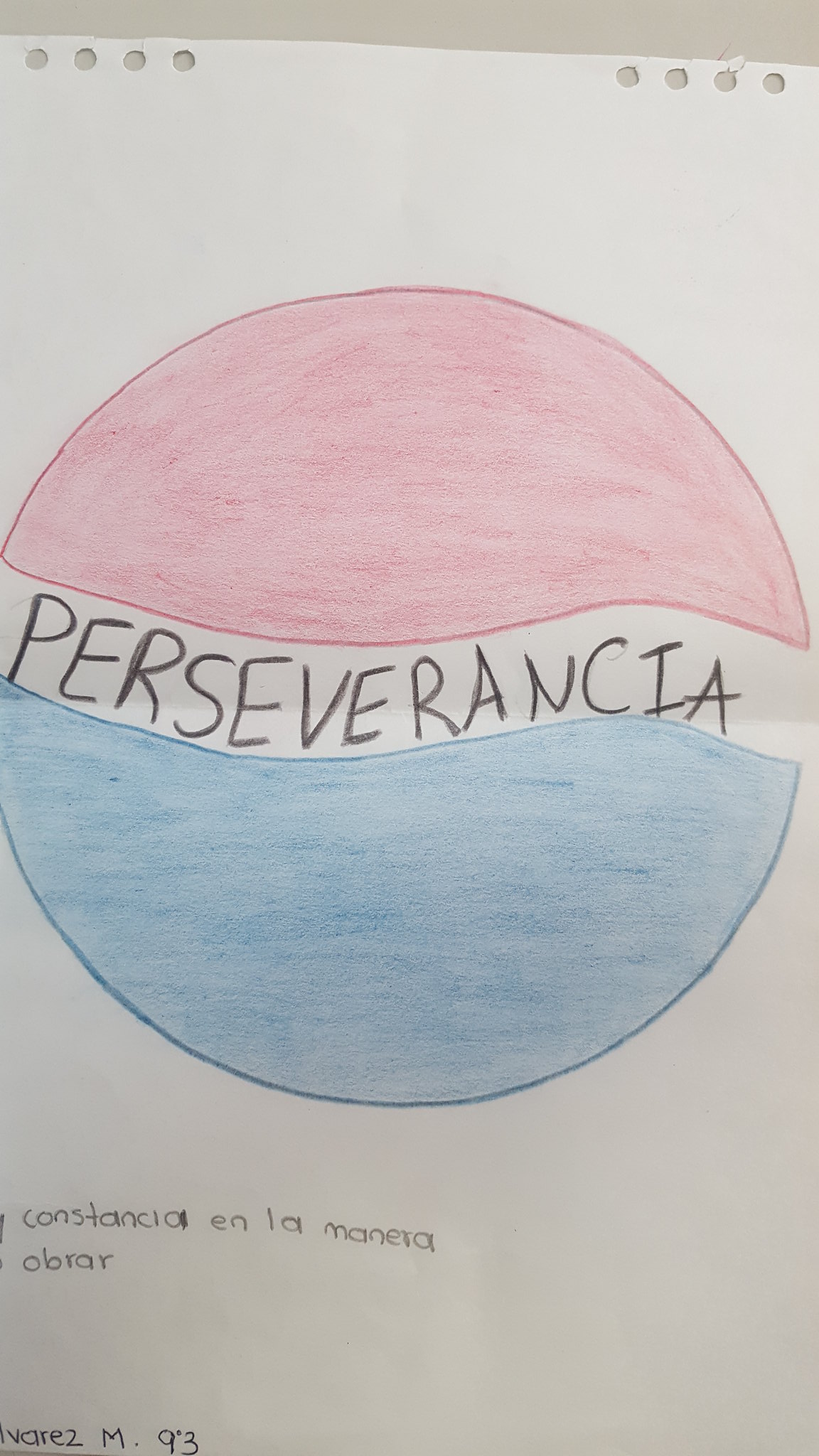This is a detailed color photograph of a hand-drawn image on a piece of white notebook paper, which has been placed against a beige surface. The paper features four round perforations at both the top left and right edges, indicating it was torn from a spiral-bound notebook. The main focus of the drawing is a large, roughly circular shape in the middle of the page, resembling the iconic Pepsi logo. The top half of the circle is shaded red, the bottom half is shaded blue, and a thin white banner with slight curvature cuts through the center, dividing the two colors.

The word "PERSEVERANCIA," Spanish for "perseverance," is dramatically inscribed in simple, uppercase black lettering atop the white banner. It appears to be handwritten with a dark pencil or pen. Additional neat handwriting in Spanish is visible towards the lower left of the page, below the drawing. This text includes what seems to be a note and a signature: "Constancia en la manera de obrar" along with the name "Alvarez M" and the date "93," possibly indicating September 3rd. The colored pencil shading displays clear strokes, and the entire page shows signs of having been folded and then unfolded before being photographed, adding to its personalized and handcrafted appearance.